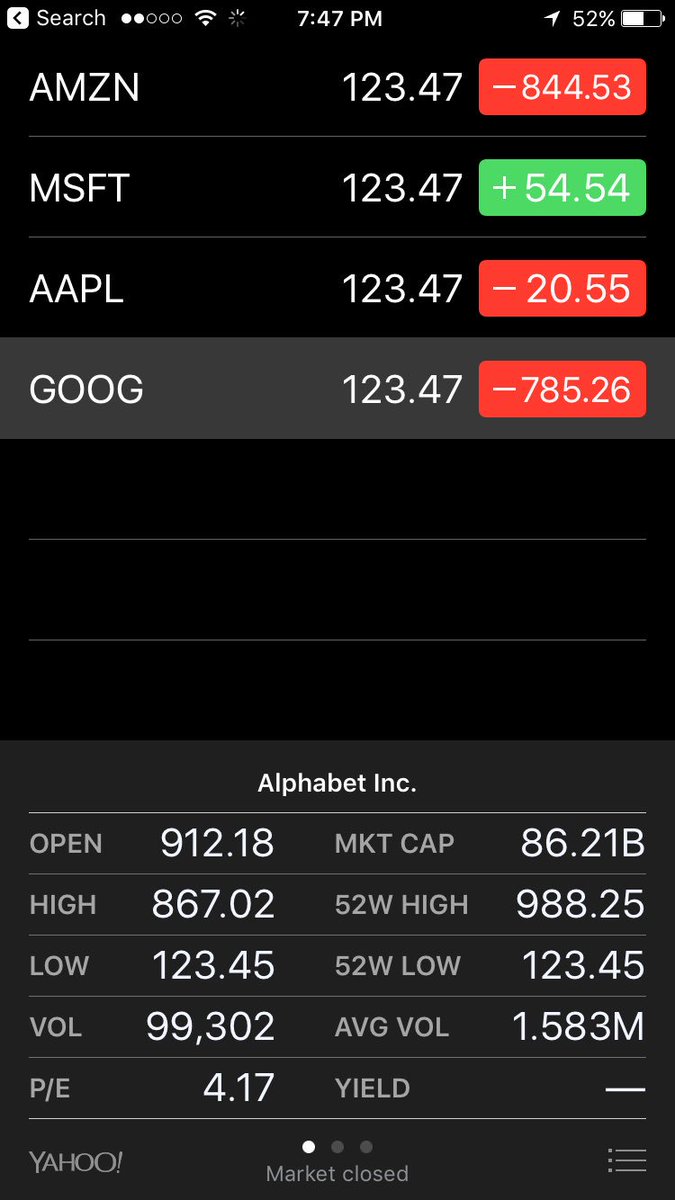Screenshot of a smartphone screen displaying stock market information with a black background. At the top, a search bar with a small white arrow inside a white box is visible, alongside two white and three black dots, indicating navigation points. The status bar shows a Wi-Fi signal icon, a cellular signal icon, the time (7:47 PM), a right arrow, a battery percentage (52%), and a battery icon.

Below, stock tickers and their respective details are listed: 
- **AMZN (Amazon)**: $123.47, down by $844.53 (in red).
- **MSFT (Microsoft)**: $123.47, up by $54.54 (in green).
- **AAPL (Apple)**: $123.47, down by $20.55 (in red).
- **GOOG (Google)**: $123.47, down by $785.26 (in red).

Following a few blank spaces, detailed information for **Alphabet Inc.** is provided:
- **Open**: $912.18
- **Market Cap**: $8621B
- **High**: $867.02
- **52-Week High**: $988.25
- **Low**: $123.45
- **52-Week Low**: $123.45
- **Volume**: 99,302
- **Average Volume**: 1.583M
- **P/E Ratio**: 4.17
- **Yield**: Not available

The bottom section includes the Yahoo Finance logo, three dots indicating more options, and a menu bar, with the market status noted as "Market Closed."